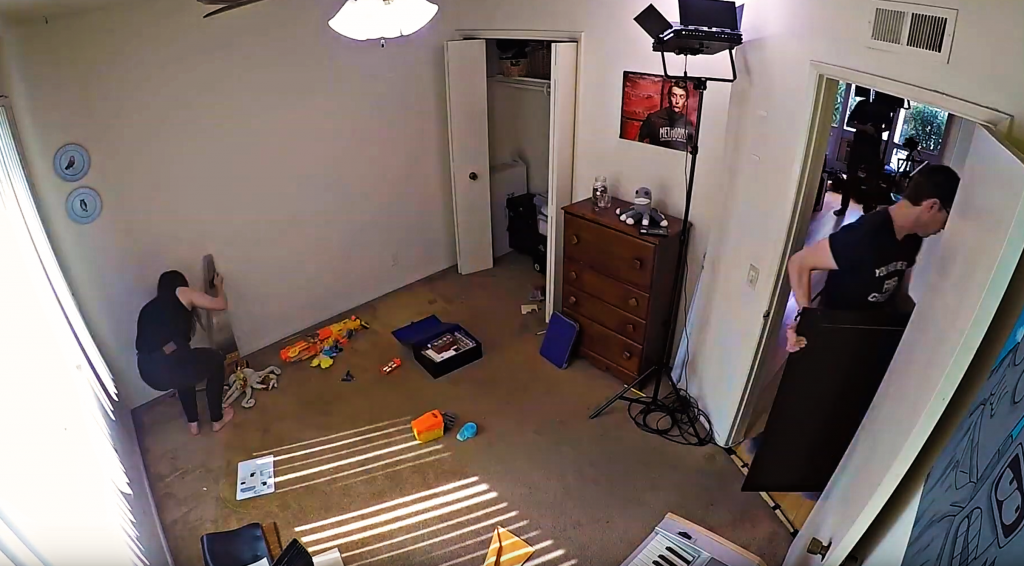The photograph, captured with a wide-angle lens, showcases an indoor room with its corners subtly curved, emphasizing the spaciousness of the area. The room appears to have white walls, albeit dirtied, and is covered in a worn, brown carpet. Diagonal lines of sunlight, filtered through the blinds, decorate the carpet. The scene suggests a period of transition, either someone moving in or out, with various items scattered around.

In the far left corner, a woman is bent over, focused intently as she holds up a saw with its blade visible. A toolbox with assorted tools lies open on the floor beside her. Directly behind her on the right is an open closet, while a small wooden chest of drawers stands nearby, adorned with a quirky sock monkey toy and a poster.

To her right, a prominent studio light illuminates the area, casting stark shadows. In the bottom portion of the image, part of a keyboard peeks into view. Beside it, a man is in mid-action, carrying a large black electronic device through the door.

In the living room in the background, another man stands near an open window, partially obscured by some unidentified equipment, suggesting he might be a musician. The photograph captures the edge of a painted mural in the lower right-hand corner, adding a splash of color and artistic touch to the otherwise utilitarian setting.